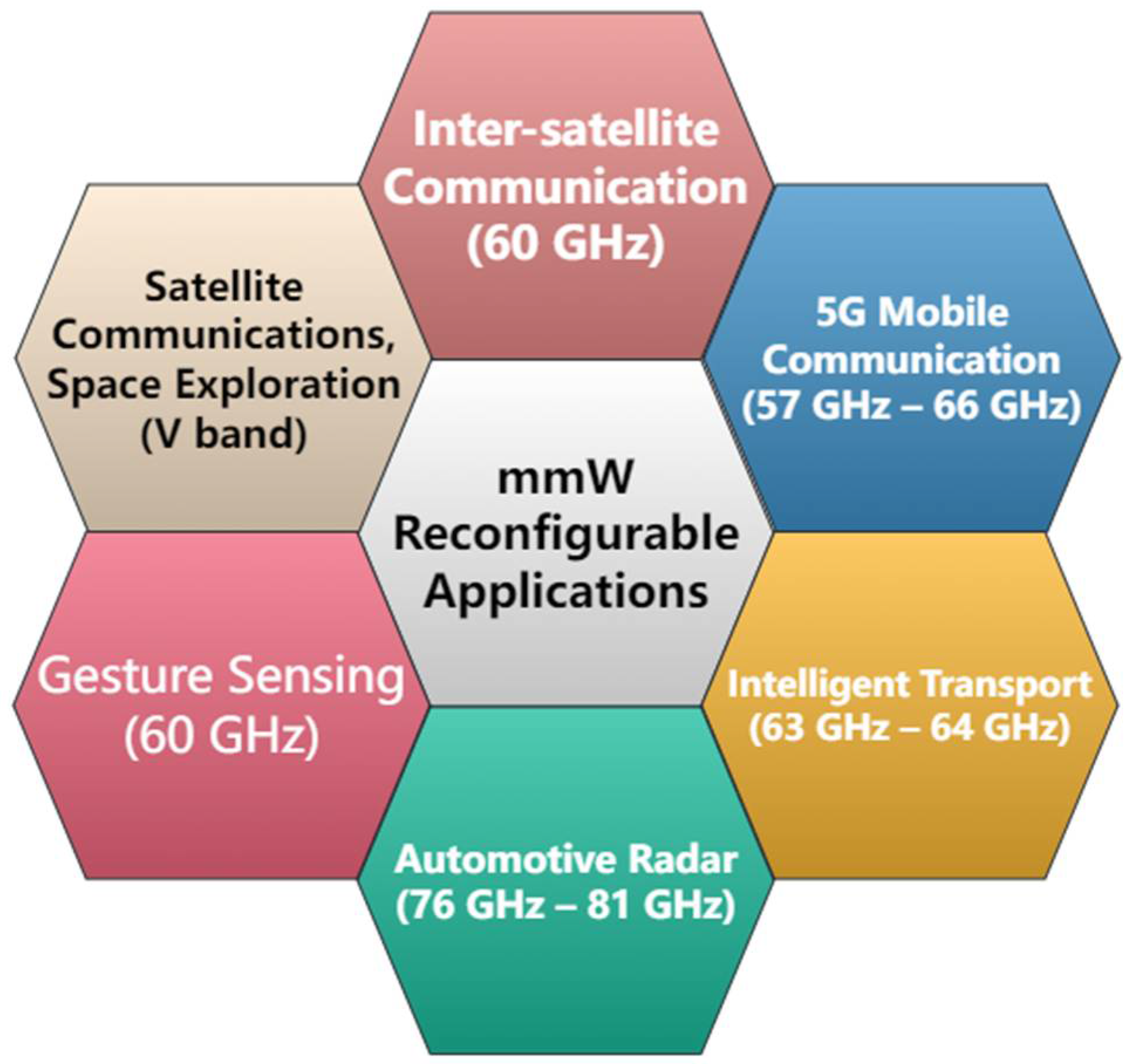The image is a detailed infographic featuring a central white hexagon with black text stating "MMW Reconfigurable Applications," surrounded by six colored hexagons, forming a honeycomb or flower-like design. Each hexagon has its own distinct color and pertinent details about different communication applications, all set against a white background.

Starting at the top, there is a pink hexagon labeled "Inter-satellite Communication, 60 GHz." To the right of this, a blue hexagon reads "5G Mobile Communication, 57 GHz to 66 GHz." Below this, an orange-gold hexagon indicates "Intelligent Transport, 63 GHz to 64 GHz." Directly at the bottom, a yellow-brown hexagon states "Automotive Radar, 76 GHz to 81 GHz." To the left, a green hexagon is labeled "Gesture Sensing, 60 GHz," and finally, at the top left, a silver hexagon reads "Satellite Communications Space Exploration, V-Band." Each colored hexagon provides specifications for different communication frequencies, creating a comprehensive overview of MMW reconfigurable applications.